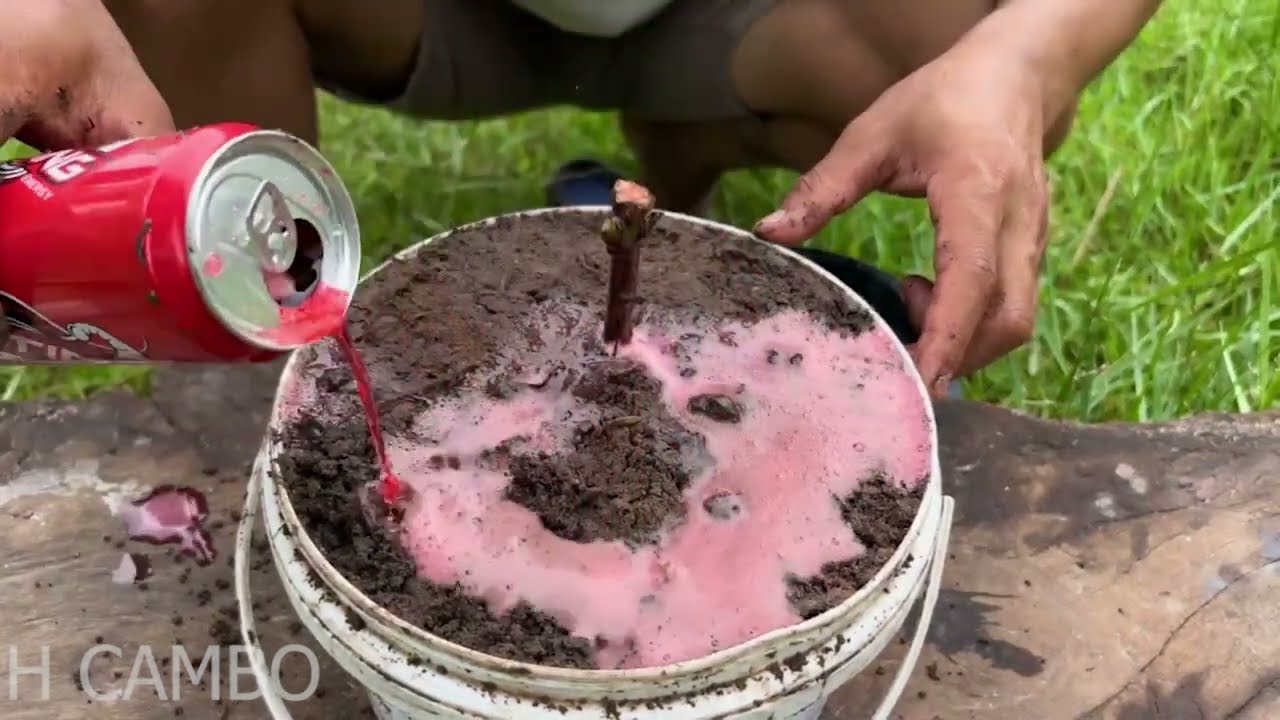A close-up view of a white plastic bucket lying on a concrete sidewalk, just at the edge where it meets a grassy surface. The bucket, dirty around the edges, is filled to the brim with a dark, almost black mud mixture, and in its center stands a stick. A person with tan skin, wearing shorts that reach the thighs, is crouched in the grass next to the bucket. This person, using their right hand for support on the bucket's rim, is pouring a can of pink or reddish soda into the mud with their left hand. The soda, possibly carbonated, forms pink bubbles on the muddy surface. The background detail includes the surface of the concrete sidewalk transitioning into a grassy area and a partially visible section of a rock that the bucket may be resting on.